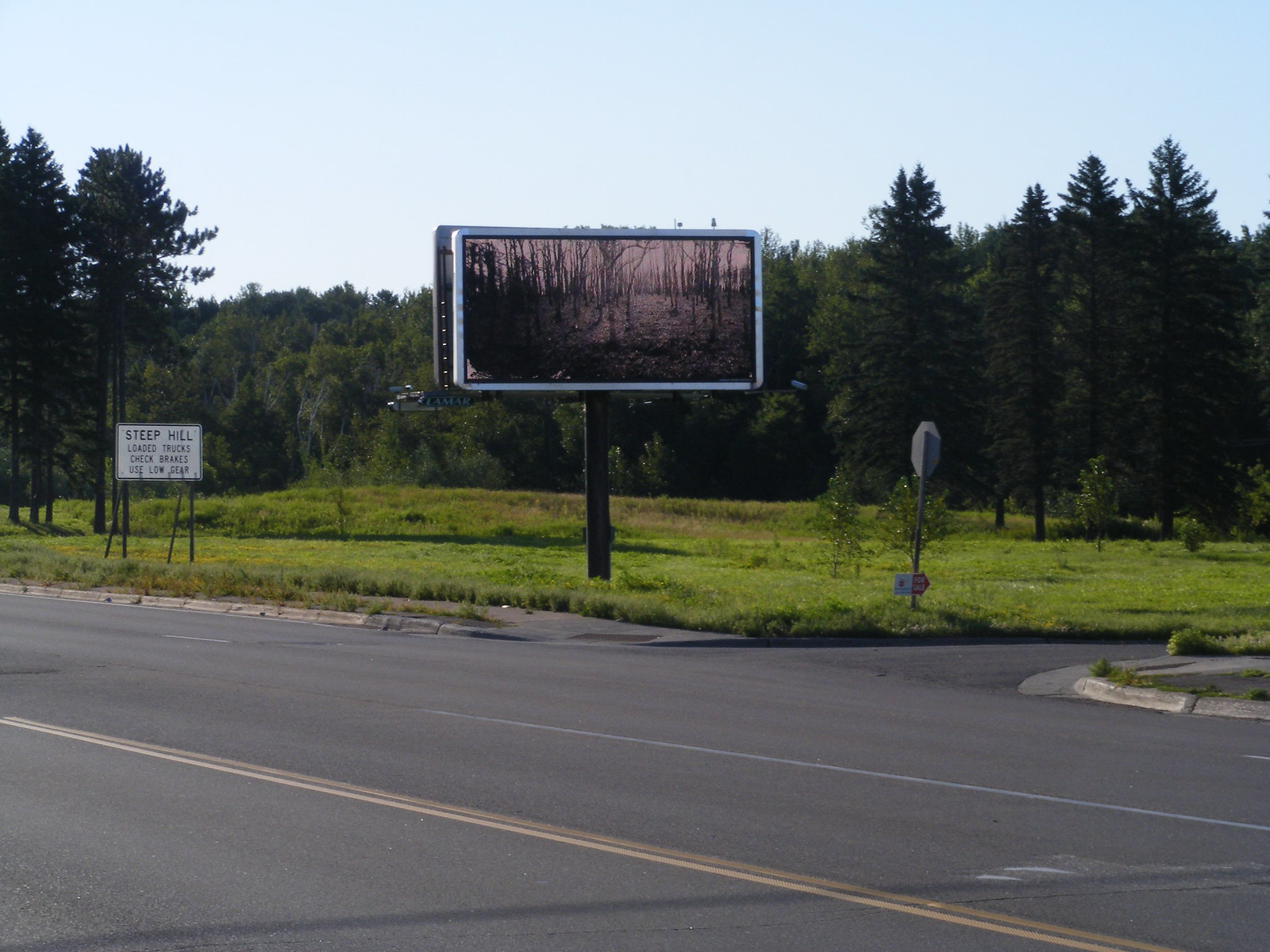This photograph captures a rural outdoor scene taken from one side of a two-lane, asphalt road looking across to the other side. Dominating the scene is a rectangular billboard mounted on a black pole anchored in freshly cut grass. The billboard features a sepia-toned image of a bare, spooky woodland, evoking a fall or winter atmosphere. To the left of the billboard, a white sign with black text warns, "Steep hill. Loaded trucks. Check brakes. Use low gear." To the right, the reverse side of a stop sign is visible. The surrounding area includes a field of grass, small bushes beneath the billboard, and a mix of fir and other trees in the background, suggesting a slightly hilly terrain. The vicinity appears relatively quiet, with no vehicles or people present, and includes sidewalks along the sides of the road.